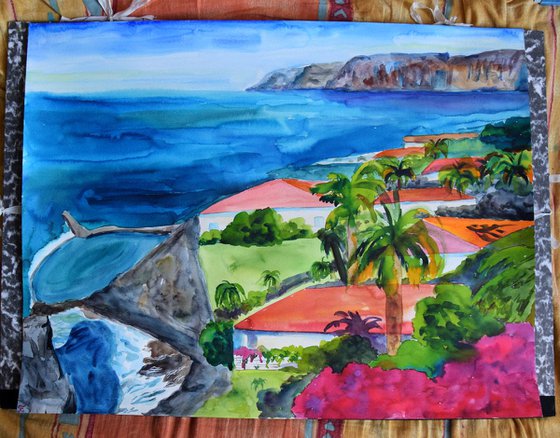The image is a detailed photograph of a vivid watercolor painting depicting a coastal, tropical village scene. The left side of the painting showcases the ocean, with high rock cliffs and outcroppings extending into the water. On the right, there is a picturesque village with houses featuring red roofs and white siding, arranged in a cookie-cutter fashion. The village is adorned with lush greenery, including palm trees, creating a vibrant tropical environment. At the bottom right, there are striking red flowers resembling fuchsia or azaleas, adding a burst of color to the scene. The entire watercolor painting is set against a black and white marbled background. This marbled background lies on a reddish-brown fabric, which has visible crinkles and folds, providing an additional layer of texture to the overall presentation. The photograph captures the vibrant details and dynamic composition of the painting, portraying an idyllic coastal village by the sea.